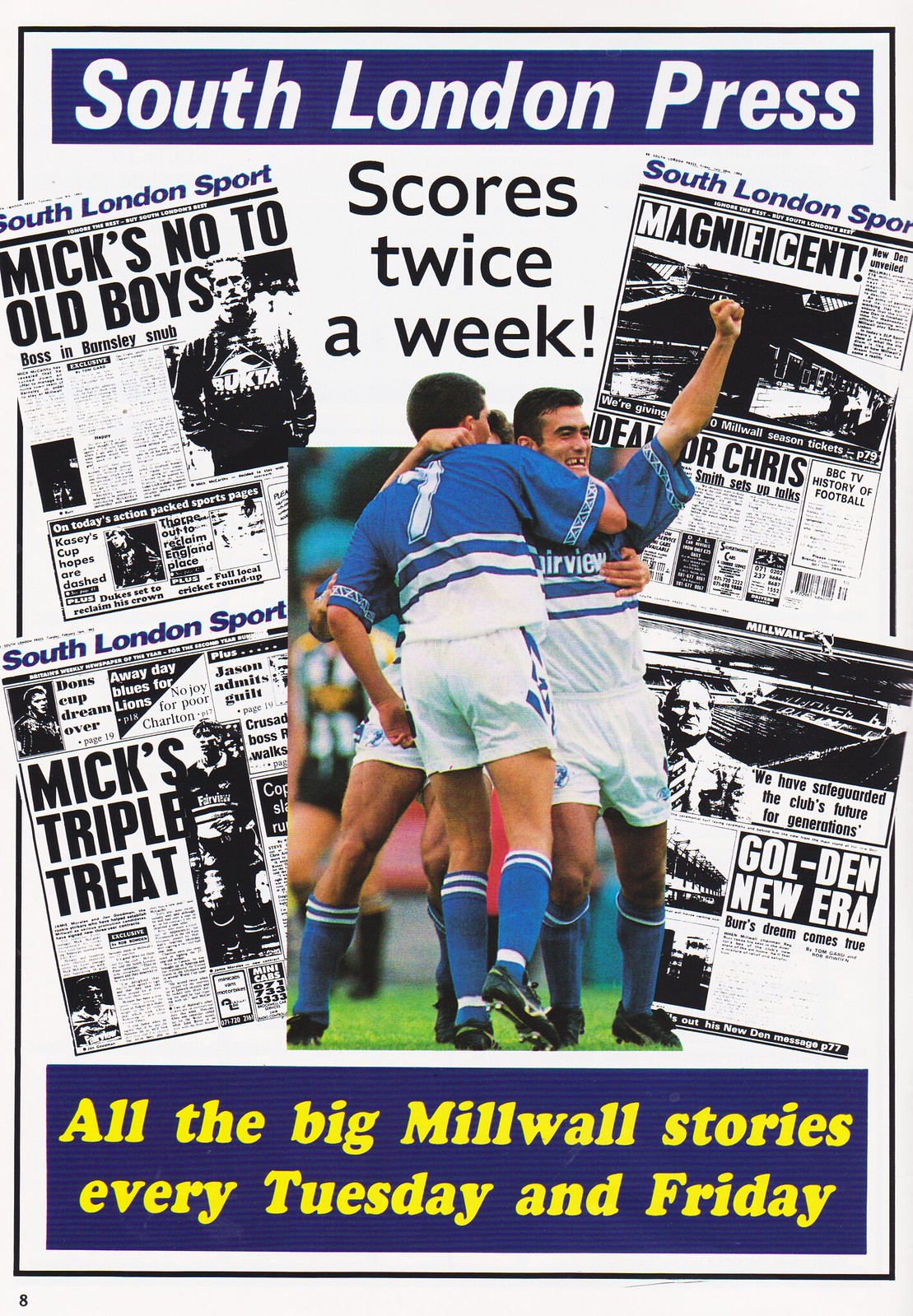The image appears to be an advertisement for a bi-weekly soccer newspaper called the "South London Press." Dominating the center of the image, a group of jubilant soccer players clad in blue and white striped jerseys, white shorts, and matching blue and white socks are seen passionately embracing and celebrating on the pitch, likely after scoring a goal. One player, prominently positioned on the right, is raising his left fist in the air while his other arm wraps around a teammate with the number 7 on his back, who is facing away from us. Notably, this player is missing a tooth, adding a touch of spirited authenticity to the scene. Their euphoria is mirrored by the presence of a referee in the background, emphasizing the authenticity of the moment.

Flanking the celebratory players on either side are clippings of various past issues of the newspaper. These clippings feature bold headlines such as "Mix No To Old Boys," "Mix Triple Threat," "Magnificent," and "Golden New Era," each adding an element of journalistic excitement to the visual experience. At the top of the advertisement, a prominent blue and white banner proudly declares "South London Press" in striking white letters. Just underneath, additional black text announces, "Scores twice a week!," enhancing the dynamic and frequent nature of the newspaper's soccer coverage.

Finally, anchoring the advertisement at the bottom, a blue banner with vibrant yellow text declares, "All the big Millwall stories every Tuesday and Friday," informing potential readers of the newspaper's regular release schedule and its dedication to covering Millwall FC.